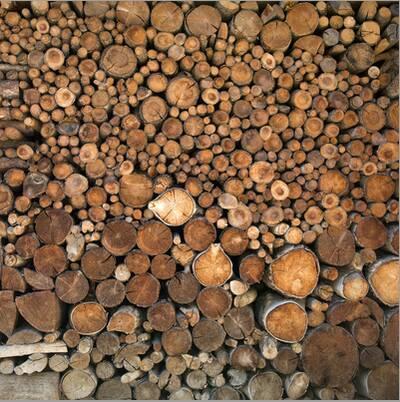The image depicts a dense stack of tree trunks cut and arranged tightly together, filling the entire frame. The trunks vary in size, with the largest ones positioned predominantly in the lower third of the square photo, gradually giving way to smaller and more irregularly shaped sections as you move upward. Among the predominantly light and dark brown logs, there is a notable exception: a whitish trunk lying on its side towards the bottom left corner. The composition, although complex and seemingly chaotic, forms a visually pleasing pattern. The color palette transitions from gray tones at the base through various shades of brown—including rich honey and reddish hues—culminating in darker tones towards the center. The textured rings inside the cut ends of the logs are prominent, revealing the intricate patterns of growth rings.